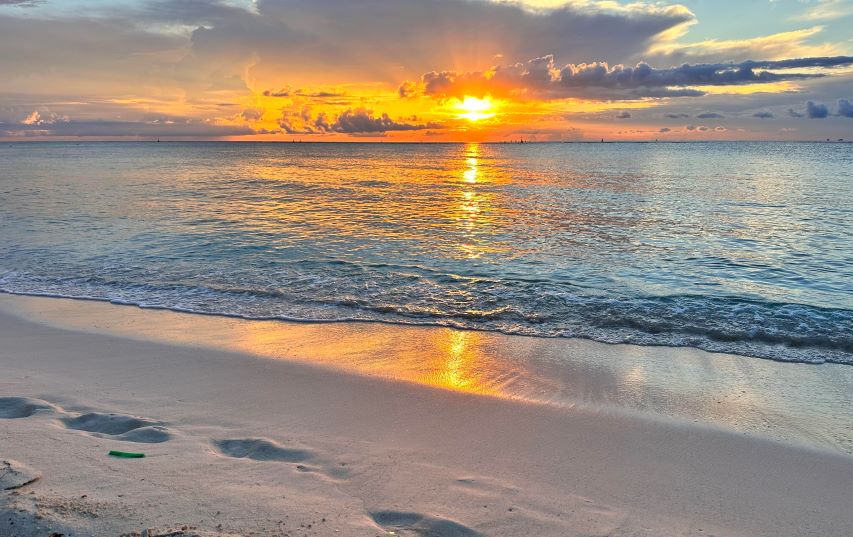This serene beach scene captures the tranquil beauty of a sunset. The sky is adorned with a mix of big puffy white clouds and darker gray-blue clouds beneath, through which a bright orange sun is emerging. The sun's rays fan out dramatically from behind the clouds, casting a golden hue across the sky and reflecting brilliantly on the ocean water, which is calm with gentle waves lapping against the shoreline. The shoreline itself bears witness to recent activity, with several footprints trailing in one direction across the smooth, pristine sand. In the distance, a few sailboats are visible against the expansive backdrop of blue skies to the right and clouds to the left, adding to the picturesque and peaceful setting. A small piece of trash disrupts the otherwise immaculate scene, reminding viewers of the human impact on nature.